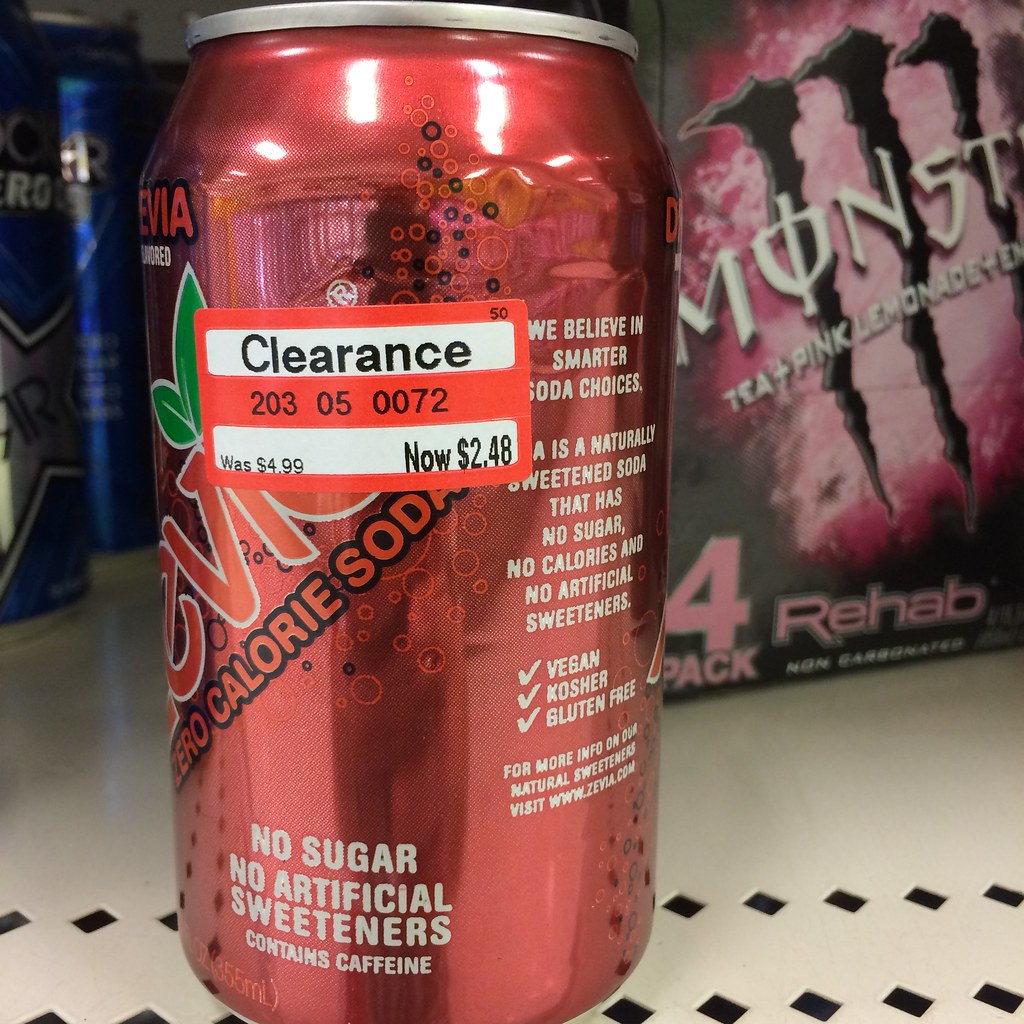The image showcases a close-up view of a metal retail shelf with square cutouts along the bottom edge, featuring two main objects. The foreground is dominated by a red can of Stevia, a zero-calorie soda sweetened with Stevia instead of sugar. The can, emblazoned with the message "We believe in smarter soda choices," also lists features like "no sugar" and "no artificial sweeteners" and contains caffeine. A large clearance sticker on the can indicates a reduced price of $2.48 from its original $4.99. The high-gloss surface of the can reflects the person taking the picture and the store environment behind them. In the background, slightly blurred but still visible, is a four-pack of pink Monster Rehab energy drinks, distinguished by their iconic slash logo.